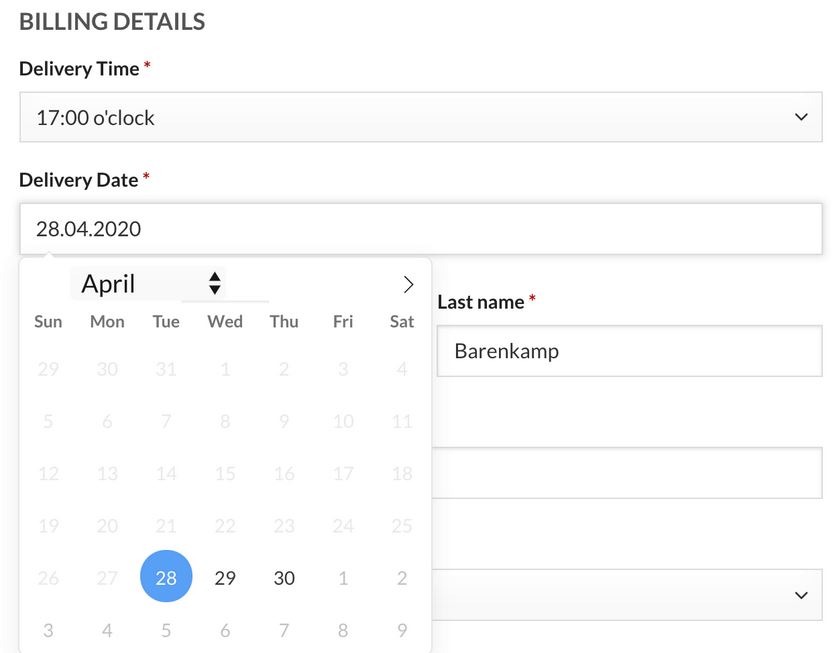The image appears to be a digital screen capture featuring an online form with billing and delivery details. The background is white with prominently displayed black text. At the top of the form, the header reads "Billing Details."

Next, there is a section labeled "Delivery Time" accompanied by a red asterisk, indicating it is a required field. A pull-down box shows "17:00" (5:00 PM) as the selected delivery time. Below this, there's another required field labeled "Delivery Date" also highlighted with a red asterisk. In this section, a white input box displays the date "28.04.2020." Beneath this input box, a digital calendar widget is visible, demonstrating the detailed date selection process.

The calendar widget shows the month of April with navigation arrows for previous and next months, and it displays the days of the week from Sunday to Saturday. All dates prior to April 28th are grayed out, indicating they are not selectable. The date "28" is circled in blue, highlighting it as the chosen delivery date. The days following the marked date, the 29th and 30th, are in black, showing they are selectable.

Further down the form, the next field is labeled "Last Name" and includes another red asterisk signifying it's a mandatory field. The entry provided is "Barenkamp" (B-A-R-E-N-K-A-M-P). Just below this, there appears to be another white input field obscured partially by the calendar widget, making its details indiscernible.

At the bottom of the form, there's another visible pull-down menu marked by a black arrow, although the field’s specific purpose is unidentified due to the limited visibility.

The text is in a large, easy-to-read font, with no additional images or noteworthy content present in the image beyond what has been described.